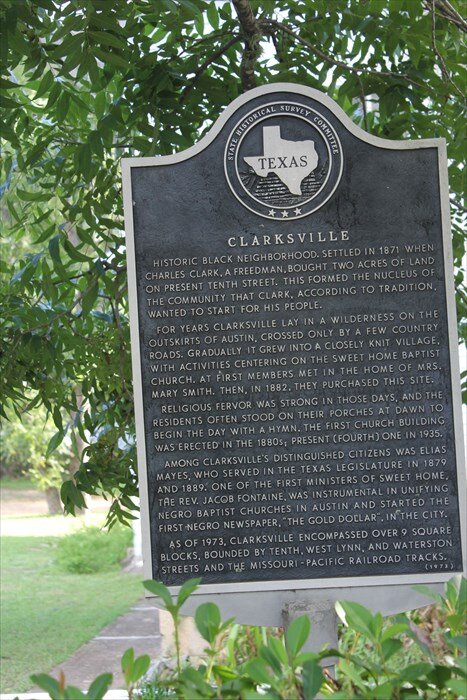This photograph captures a historical marker under a lush, leafy tree with vibrant green grass, suggesting it is spring or early summer. The marker prominently features the seal of the State of Texas at the top. This plaque, from the Texas State Historical Survey Committee, commemorates Clarksville, a historic black neighborhood established in 1871 when Charles Clark, a freedman, purchased two acres of land on present-day 10th Street. This marked the beginning of a community Clark intended to create for his people. Initially lying in the wilderness on the outskirts of Austin, crossed only by a few country roads, Clarksville gradually grew into a closely-knit village centered around the Sweet Home Baptist Church, which began in the home of Mrs. Mary Smith and moved to its current site in 1882. Residents, driven by strong religious fervor, often started their day with hymns sung from their porches. The historical marker gives further details about the town's small size and its development, indicating the community's rich heritage and historical significance. To the side, a sidewalk can be seen, suggesting that this location now serves as a site of interest for visitors.